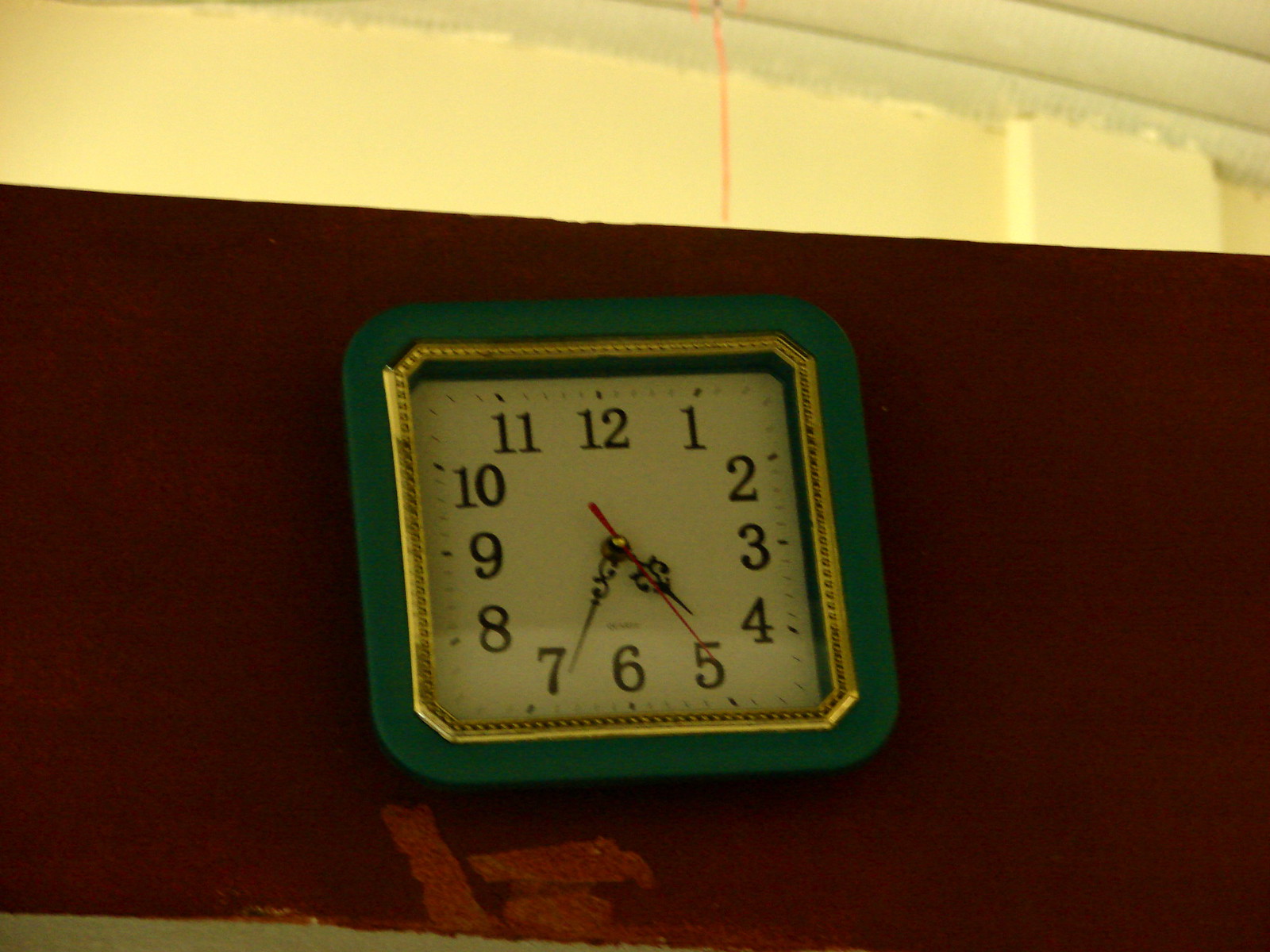A close-up photograph captures a square-shaped wall clock resting on dark red fabric, with a white wall serving as the backdrop. The clock's frame is dark green with a subtle gold inner line, offering a rich contrast. The clock's face is off-white, adorned with black numbers and time notches. The hour and minute hands feature an elegant swirl design in black, while the long seconds hand stands out in red. The time displayed is 4:34, with the seconds hand precisely on the 5-second mark.